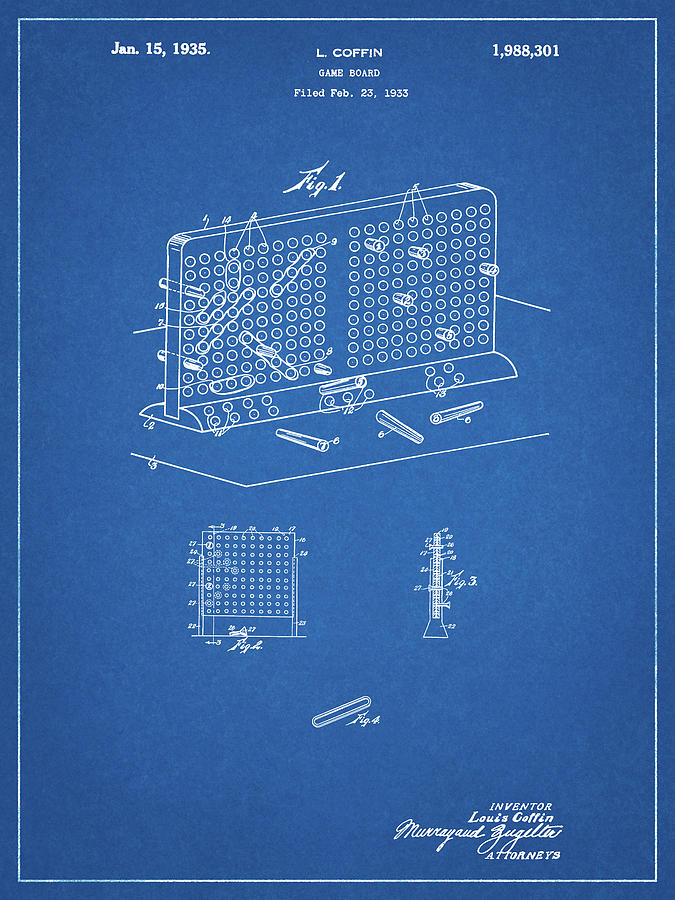This detailed diagram, set against a blue background, is rectangular with a prominent thin white line bordering its interior. Toward the upper center is a horizontal rectangle containing two squares, one on the right and one on the left, each formed by an outline of small, perfectly aligned white circles. The base of this rectangle curves slightly over the front, drawing attention to its structure. Below this, there is a single square, appearing as a continuation of the ones above, also outlined in white and filled with an array of small white circles. Anchoring the diagram at the bottom center is an oblong white shape accompanied by diminutive white text situated to its right, completing the intricate and visually engaging schematic.